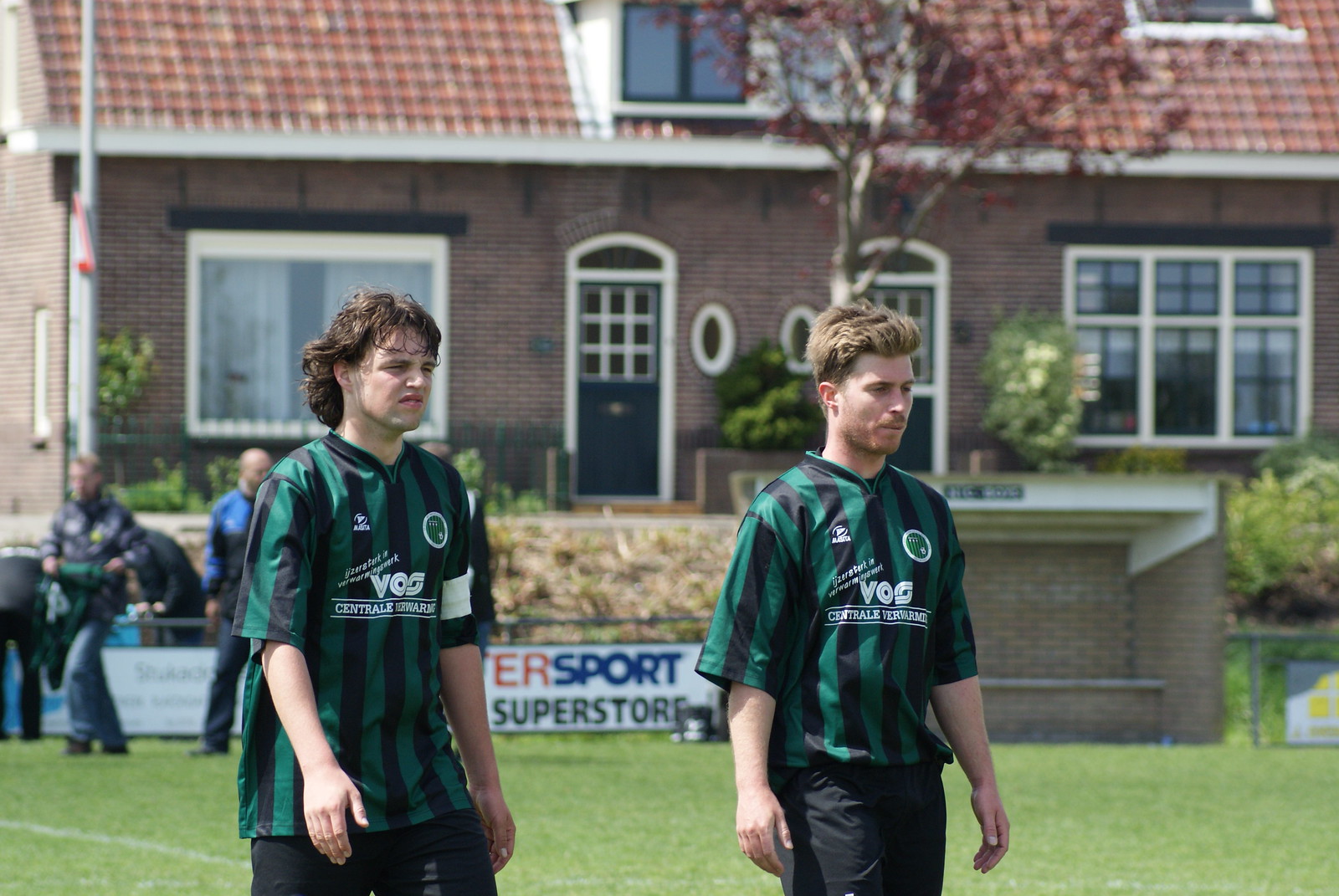This photograph captures two male athletes standing side by side on a grassy field. Both are dressed in matching black and green striped jerseys adorned with white lettering. Their lower attire—whether black pants or shorts—is indistinct, and their arms rest nonchalantly by their sides. Behind them, the lush greenery of the field is visible, along with the corner of a brick structure to the right of the athlete on the right. In the background, two additional figures are present, although details about them remain unclear. Between the two primary athletes, a sign partially emerges, displaying the words "ER SPORT SUPERSTORE" on a white banner. Further in the distance, there’s a brick house characterized by a dark-colored door at its center, a similar door to its right, and large windows flanking both doors. A tree stands in front of the house, which features a red shingled roof.